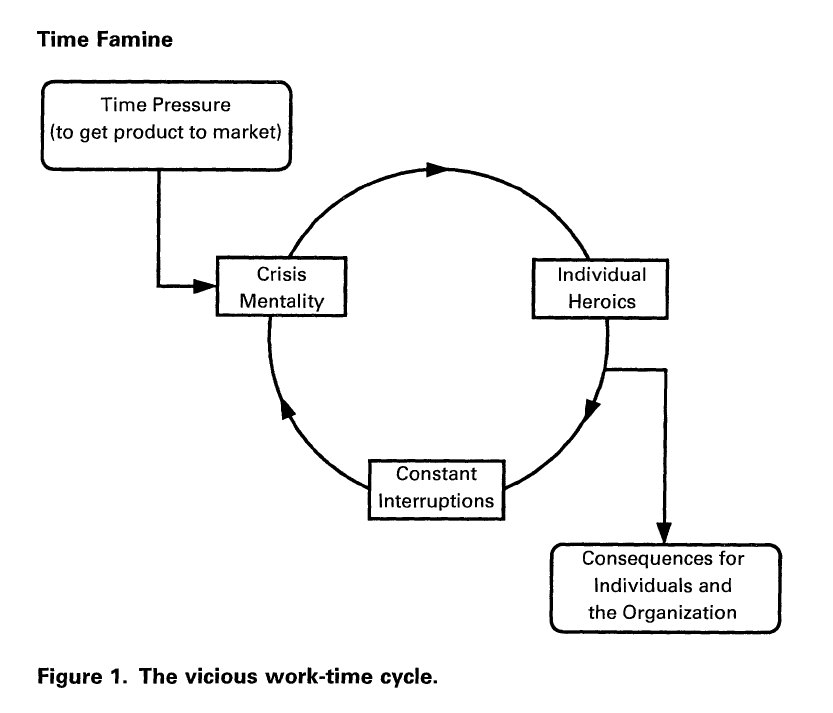In this image, a detailed chart titled "Figure 1: The Vicious Work-Time Cycle" is displayed against a plain white background with black text. The diagram, which resembles a scanned document or slideshow presentation, highlights a cyclical pattern of workplace challenges. In the upper left corner, the term "Time Famine" is prominently featured. Below that, a rectangle labeled "Time Pressure to Get Product to Market" transitions via an arrow into another rectangle titled "Crisis Mentality." This crisis mentality is encapsulated within a circular flow that includes "Individual Heroics" on the right side and "Constant Interruptions" at the bottom. An arrow from the circle's right side leads downward and outward to another rectangular box labeled "Consequences for Individuals in the Organization." The chart uses straightforward black text and simple arrow lines to illustrate the interconnected and repetitive nature of these work-related issues.